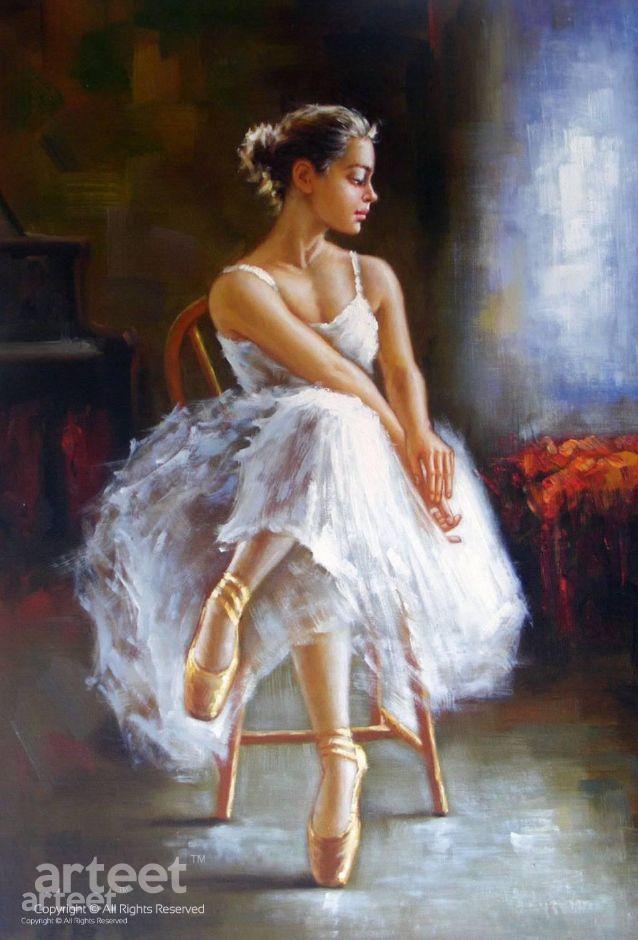This detailed painting captures a serene ballerina seated elegantly on a wooden chair. The ballerina, dressed in a poofy white ballet dress, has her dark hair neatly up in a bun and is wearing golden ballet shoes. Her posture is relaxed yet poised, with one leg crossed over the other; her right foot rests on the floor while her left foot is placed above it. She looks off to the right, presenting a calm, side-profile view, with her hands gently resting together towards her right side. 

The background is split into two distinct color tones: a yellow-brown hue on the left side and a bluish tint on the right. On the left, the edge of a grand piano is visible, adding a touch of sophistication to the setting, while a reddish object can be faintly discerned on the right. The environment, though understated, complements the ballerina's tranquil demeanor. At the bottom left corner of the image, the word "A-R-T-E-E-T" is marked, signifying the artist’s signature.